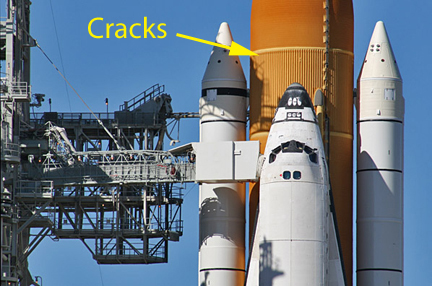This photograph captures a space shuttle preparing for launch. The shuttle occupies the right portion of the image, while the left half is dominated by a silver-gray metal scaffolding that forms part of the launch support structure. The visible section of the shuttle includes the nose cone, where the flight crew would sit, alongside partial views of the large orange central fuel tank and the two white booster rockets flanking it. The solid blue daytime sky serves as the backdrop for the scene.

A key feature in the image is a yellow label near the top left corner, displaying the word "Cracks" with a capital C followed by lowercase letters. An arrow extends from this text, pointing towards the orange fuel tank above the nose of the shuttle, indicating specific areas of concern. Although the image quality is low, resulting in an unclear view of the cracks, the label and arrow emphasize their location. The structure remains grounded and stationary, firmly attached to the metal platform, with no people visible in the scene.